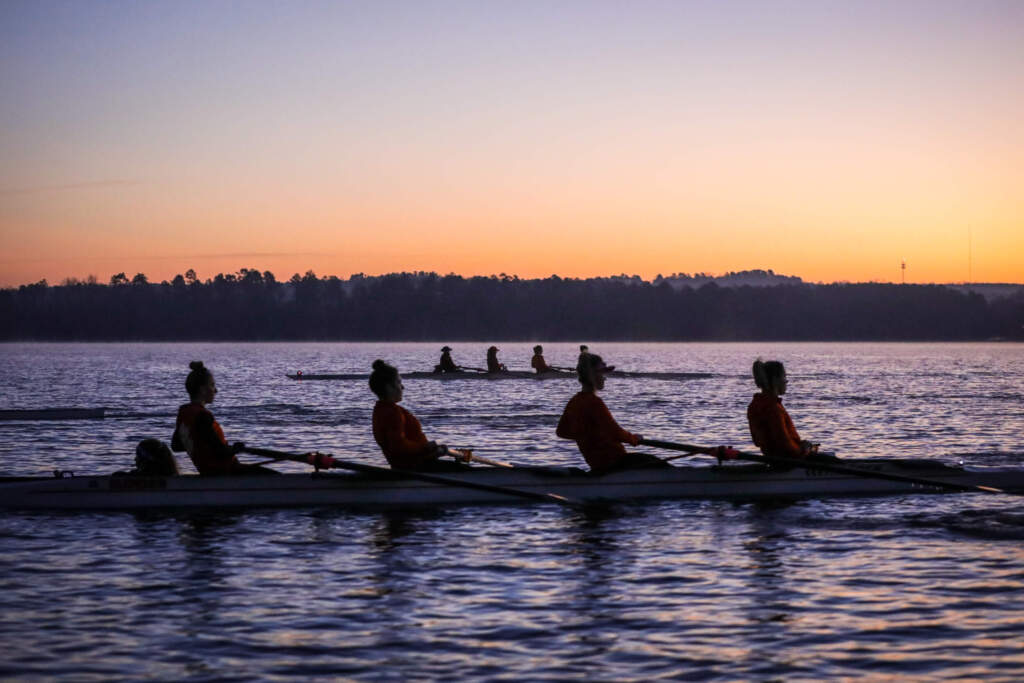This photograph captures a serene scene likely at dusk, featuring two long canoes gliding across a large, calm body of water—possibly a river or lake. The sky is a gradient of orange and yellow near the horizon, transitioning to a hazy blue at the top, reflected beautifully on the dark water. The water shows subtle ripples caused by the rowers' paddles.

Each canoe, low in the water, holds four rowers seated sequentially, their outlines faint in the dim light. The rowers in the foreground are identifiable as women with hair tied in buns, wearing long-sleeved red shirts or jackets, rowing in unison with their oars extending out to the sides. The second canoe, further back, trails in the same direction, emphasizing the rhythmic synchronicity of this competitive rowing event, akin to the sport of crew.

In the background, silhouetted against the twilight sky, stands a dense forest, further shrouded in the encroaching darkness. Above this tree line, a small wooded hill adds depth to the scene. A large building is faintly visible off in the distance, contributing to the landscape's complexity and framing this tranquil, yet dynamic twilight tableau.